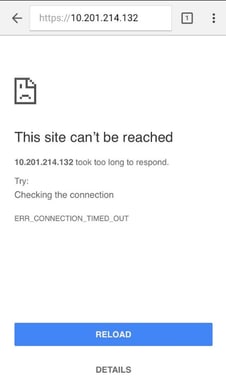This image captures a close-up of a smartphone screen displaying a web page error message. At the top of the screen, there's a gray rectangular bar with a left-pointing arrow, followed by a URL field containing the address "https://10.201.214.132". Beneath this, the main white section of the screen prominently shows the message "This site can't be reached." A distressed rectangular icon with a dog-eared corner and a frowny face sits below the message. The error explanation reads, "10.201.214.132 took too long to respond," suggesting a timeout issue. It is followed by troubleshooting advice: "Try checking the connection," and the error code "ERR_CONNECTION_TIMED_OUT." At the bottom of the screen, there is a long, skinny bluish rectangle labeled "Reload" in black print, accompanied by another option "Details" beneath it. Additionally, the top section of the screen includes a boxed number "1" and a menu represented by three vertical dots, indicating more options available for interaction.